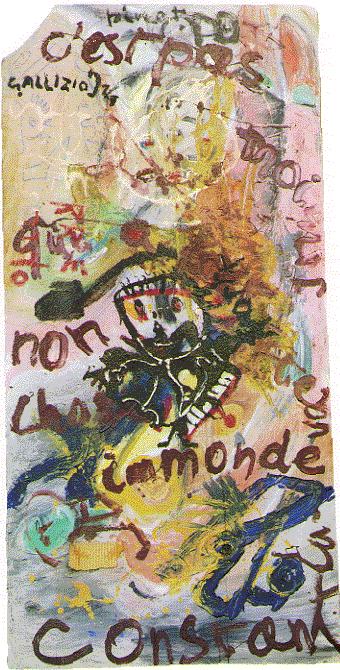The image is a vibrant and abstract painting with a distinctly eerie yet captivating style, showcasing a central skeletal face rendered in black and white. Surrounding the skeletal face are various French words, prominently including “C-E-S-T-P-A-S” at the top, “N-O-N” to the left, “I-M-M-O-N-D-E” in the middle, and “C-O-N-S-S-A-N-T” at the bottom. Additionally, scattered letters such as “J-N-T-U” are interspersed throughout the image. The skeletal head, positioned dead center, features defined eyes and a mouth, with a faint image of another face subtly present above it, accompanied by the word "C-A-L-L-I-Z-I-O" to the left.

The background is a chaotic yet visually striking mix of pink and light yellow splashes, lending a vibrant and somewhat childlike aura to the piece. The painting evokes the sense of a surrealist or avant-garde poster, possibly hinting at an advertising motif with its array of prominent text placements that could suggest themes like a restaurant or cafe with a musical ambiance, as inferred from the elements resembling a piano or keyboard. The lower right corner intriguingly includes a blue, rope-like figure that vaguely resembles an eye of a serpent, adding a layer of futuristic mystique to the artwork.

Combining these elements, the image presents an enigmatic blend of artistic expressions with an undercurrent of French cultural references, encapsulating a vivid and somewhat disconcerting tableau.